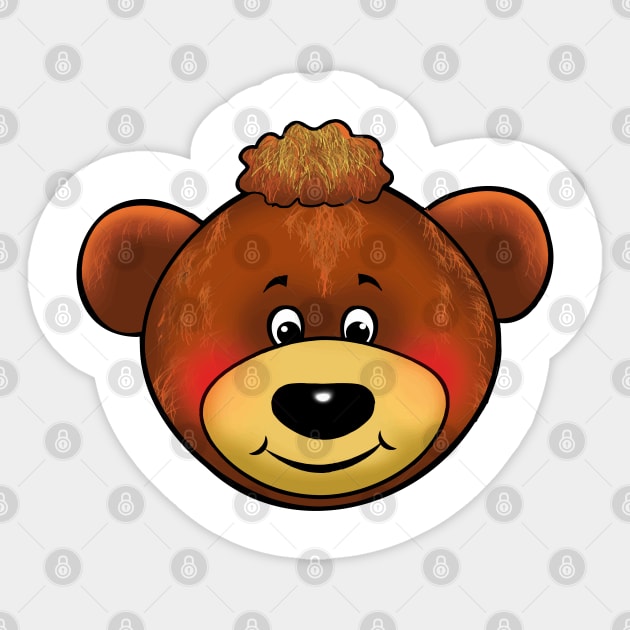This rectangular, horizontal image features a cartoon bear at its center. The background is predominantly gray with an overlay of darker gray dots and circular patterns, emphasizing depth and texture. The bear, positioned centrally, has a charming, oval-shaped head topped with a tuft of fluffy hair. His ears are brown, matching his dark brown body, while the area around his nose and mouth is a lighter brown. His facial features are detailed: he has two expressive eyes, a big black nose, and a small smiling mouth. The bear's hair, slightly lighter than the rest of his head but not as light as the nose and mouth area, adds to his endearing appearance. The bear is encased within a white border that prominently separates him from the patterned background. Additionally, subtle diagonal lines and watermark logos are visible throughout the image, serving as a form of copyright protection. The overall composition, along with the contrasting colors and patterns, highlights the bear's cheerful expression and inviting demeanor.